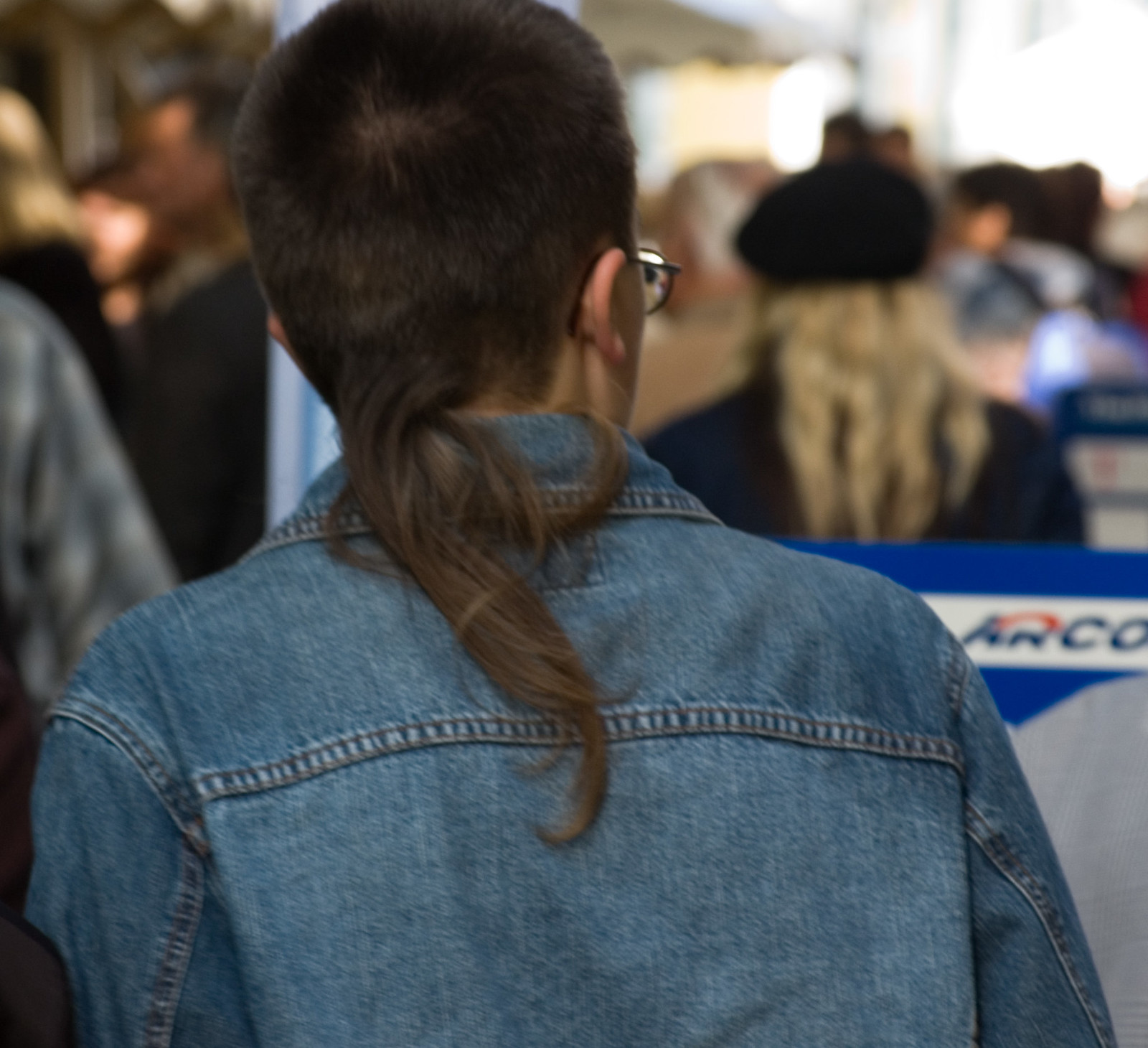In this outdoor daytime photo, the focus is a young man with short, darker colored hair styled in a mullet, where the hair is very short on top and extends long past his shoulders at the back. He is wearing black glasses and a blue jean jacket. The picture is taken from behind, showing him facing away and slightly to the right, revealing his ear and the side of his face. The background is blurred, populated with several people, including a woman with long blonde hair wearing a black coat and a black hat to the right, and a gentleman in a plaid outfit to the left. Behind them, a blue and white partition displays the word ARCO in blue letters on a white background.